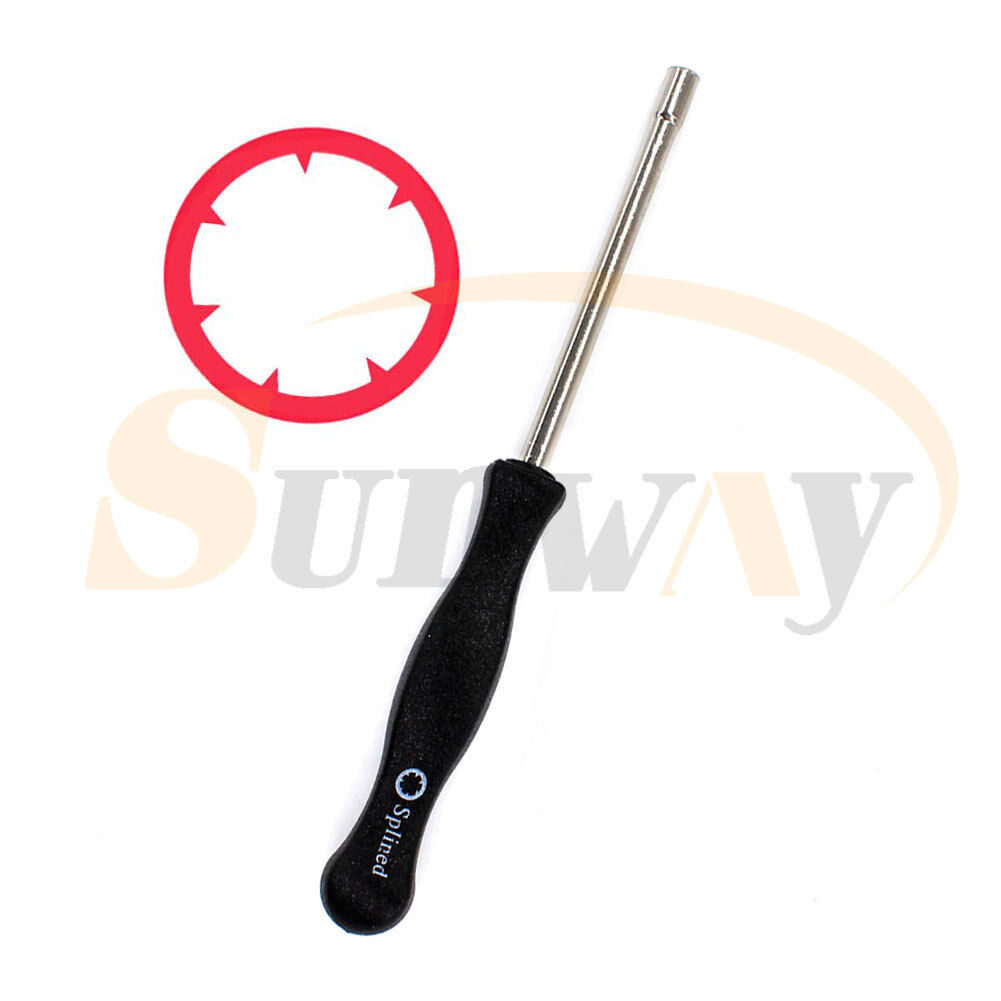This product photo showcases what appears to be a precision hand tool, likely a specialized screwdriver, against a white background. The tool features a black handle with white text that reads "Splined" and is accompanied by a distinctive logo that resembles a bolt. This logo also appears enlarged and in red to the left of the tool. The handle attaches to a metallic rod which terminates in a tip designed for fastening or loosening bolts. In the background, the word "Sunway" is lightly printed in a semi-transparent, almost watermark-like fashion, with the 'S' and 'A' highlighted in yellow. Above the "Sunway" text, there is a yellow curve ending in a red circle fringed with seven small triangular spikes.